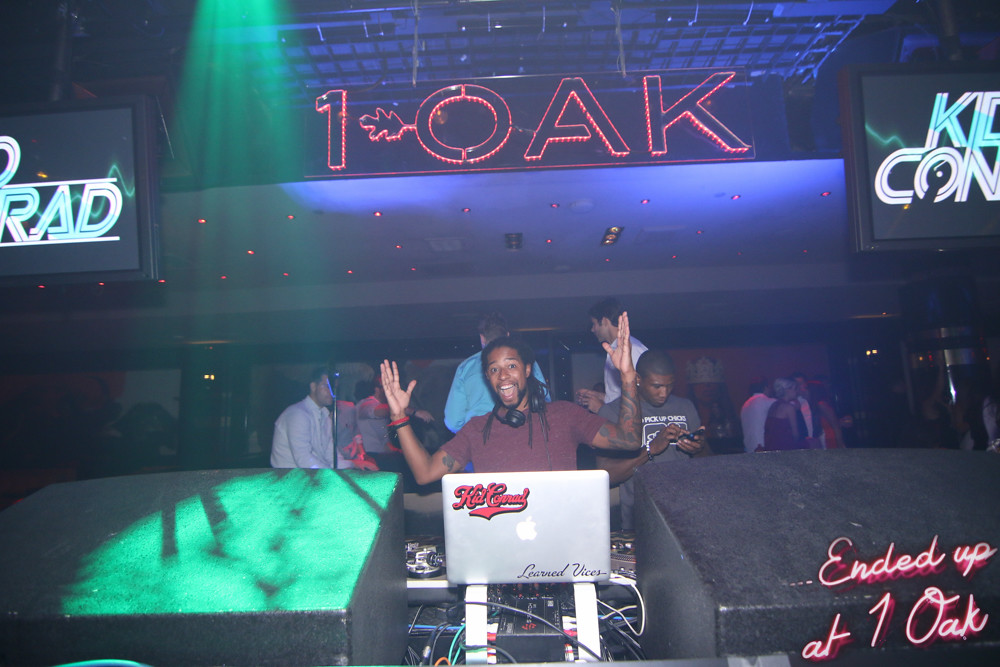This photograph, taken indoors in a vibrant nightclub, captures an energetic DJ moment. Dominating the top center of the image, a neon sign spells "1 OAK" with an oak leaf emerging from the left side of the 'O'. The DJ, standing proudly in the foreground, is an exuberant figure with dreadlock-style hair and a beard, donning black headphones around his neck and wristbands on his right wrist. Both his arms are triumphantly raised, and he sports a broad smile. Positioned behind DJ equipment and an Apple laptop, he appears to be the heart of the party. Surrounding him in the background, a diverse crowd mingles and engages in various activities, including one person on a phone and a woman wearing a paper crown. Screens flanking the DJ display the text "KD Khan" or a similar name. The lighting is dynamic, with green stage lights and multiple neon signs, including one in the lower right corner that states "ended up at 1 OAK." This lively scene is emblematic of a jubilant nightlife atmosphere, encapsulating the essence of the club.